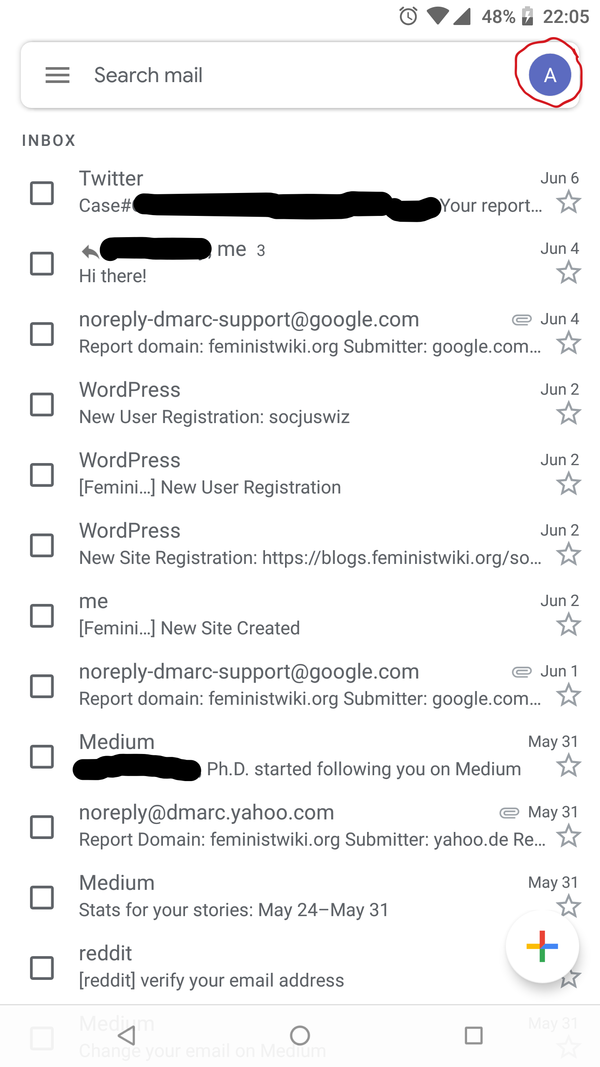The image depicts a screenshot of someone's email search results. Dominating the top right corner is a capital "A" enclosed in a purple circle, which is notably circled with a red pen, drawing attention to it. Throughout the page, several areas have been blacked out with a Sharpie, likely to obscure sensitive information.

The visible content shows various emails listed, with a timeline spanning from May 31st to June 6th. On the left side of the list, there are checkboxes beside each email, allowing the user to select them for bulk actions such as deletion. The interface includes a "Search Mail" function at the top.

Notable email entries include:
- An email with the subject line "Twitter"
- A message beginning with "Hi there"
- Multiple notifications from "WordPress" indicating new user registrations, detailed as "femini" and "cell site registration"
- Emails from "no-reply@domain", "support", and "report"
- Messages from "Medium" and "Reddit"

Beneath the "Inbox" label is a cluttered assortment of subjects and senders, indicative of a typical, busy email account with diverse sources of incoming mail.